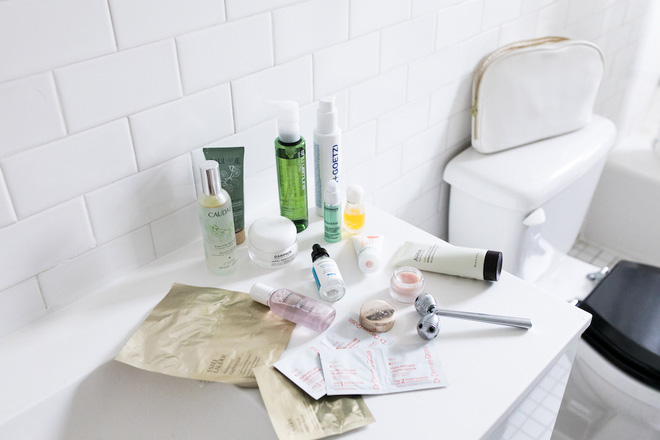The image depicts a cluttered restroom countertop laden with various self-care items. The back wall features a pattern of white, brick-shaped tiles divided by lines, providing a clean, modern backdrop. On the left side of the countertop, there are two silver packages. Moving upward, there is a bottle with a white label partially reading "CA," and behind it, another container is visible, distinguishable by its orange-colored top and upside-down position.

Next, there is a bright green bottle with a white pump top. To its right is a tall, thin white cylinder that appears to be a spray dispenser, accompanied by a small white jar with a proportionally large, round lid. Adjacent to these items is a light green, bullet-shaped container.

Following this arrangement, there is a small bottle filled with yellow liquid and topped with white, positioned next to a bottle of purple liquid that has been knocked over, causing foamy bubbles at its side. A dropper bottle with a white label and some blue detail lies on its side nearby. Further along, there is a white tube with a pink circle on its cap alongside another white tube with a black cap, also lying flat.

Additionally, there is an open jar of pink substance with its rose gold lid placed to the side. A silver stick-like object with rounded balls on each end lies nearby, next to a packet of white squares with red text.

Finally, on the far right atop a white porcelain toilet with a black seat rests a handbag, completing the snapshot of this jam-packed bathroom scene.